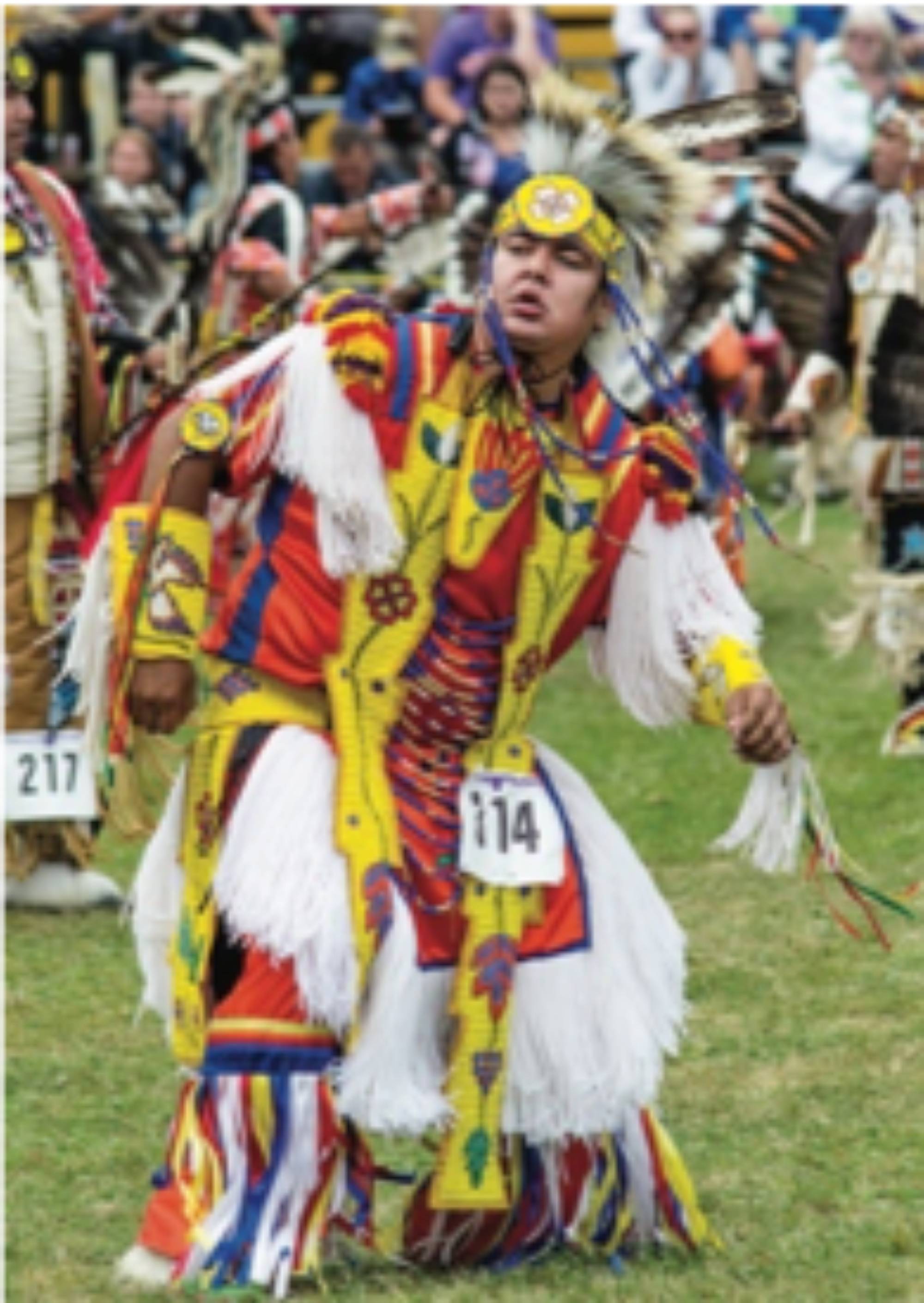The image captures a vibrant scene of a Native American dance competition set on a green grass field under daylight. The central focus is a Native American man in full ceremonial regalia, engaging mid-dance, leaning slightly to his right. He is adorned with a fur headdress featuring a large yellow band and an intricate beaded pattern. His outfit includes white fur wrapped around his shoulders and waist, resembling a skirt, with flowing fabric fringe on his legs, reminiscent of a shredded flag. He also wears a long, beaded scarf adorned with flower or leaf designs, which extends almost to the ground, and matching beaded cuffs on his forearms featuring colorful bird patterns. His competition number, 114, is prominently displayed on his outfit. In the blurred background, other participants in varied traditional attire can be seen, including one with the number 217. Spectators in everyday clothing are seated on bleachers, indicating a large, attentive audience for this cultural event. The scene’s vivid colors include dominant shades of yellow, red, blue, and white, creating a striking visual of traditional Native American craftsmanship and performance.